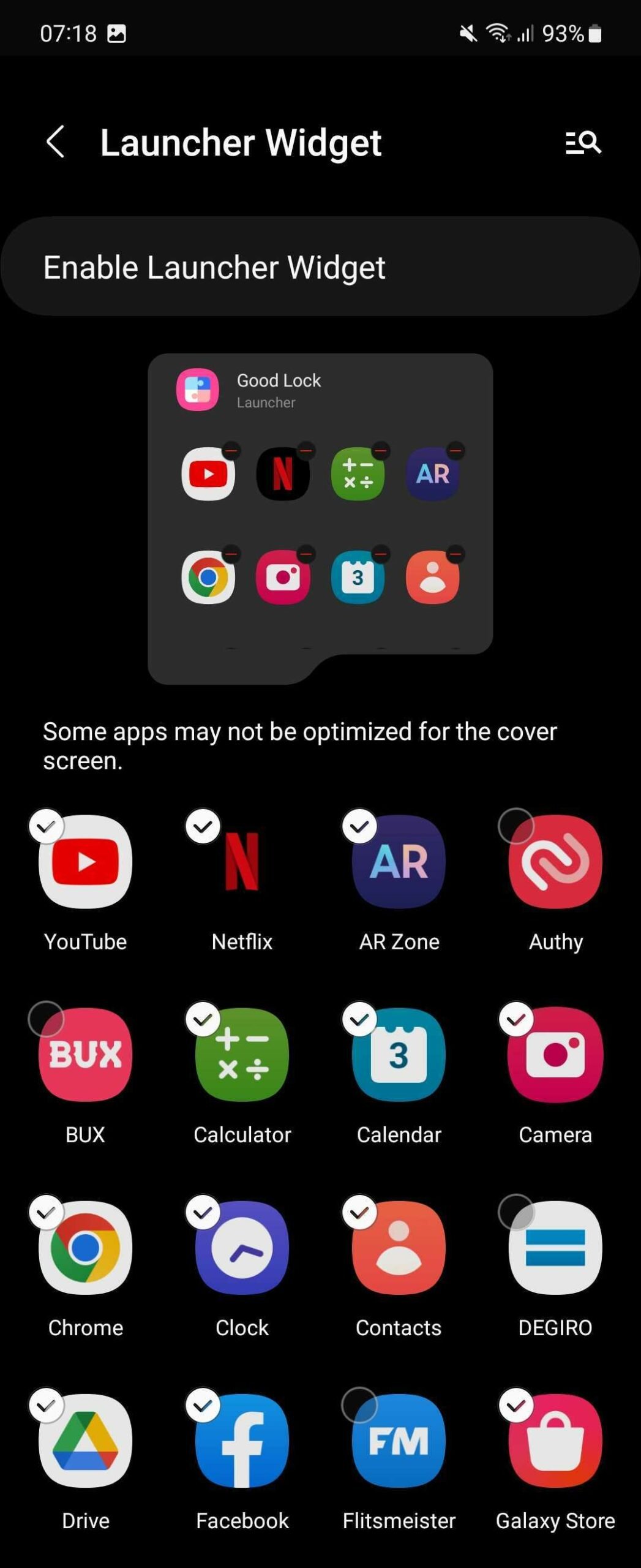This image is a detailed screenshot taken from a smartphone. The entire screen displays a solid black background. In the upper left corner, white text shows the time, "7:18," alongside an icon for gallery images. On the upper right corner, several status icons are visible: the volume and sound are muted, Wi-Fi is enabled with three out of four bars lit, and the battery icon shows a 93% charge.

Below these status indicators, large bold white text reads "Launcher Widget," with another line below stating "Enable launcher widget." Directly beneath this text lies a gray square box containing several app icons. Positioned centrally within this box are icons for YouTube, Netflix, Google Chrome, and the Calendar app.

Further down, a line of white text cautions, "Some apps may not be optimized for the cover screen." Below this warning on the left side, additional app icons are displayed in sequence: YouTube, Netflix, AR Zone, and Authy.